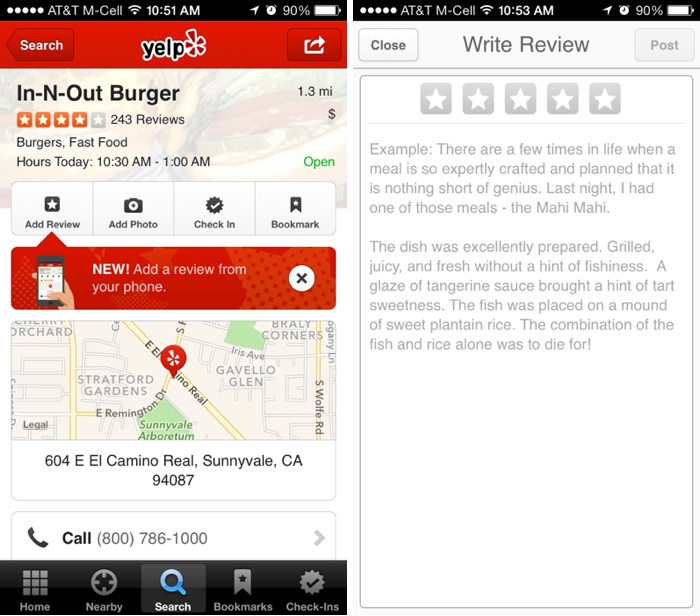The image consists of two screenshots taken from a smartphone displaying a Yelp review interface for In-N-Out Burger. The first screenshot, captured at 10:51 AM with a 90% battery level, shows the Yelp application with a red navigation bar at the top. The page is for In-N-Out Burger, located 1.3 miles away, holding a four-star rating based on 243 reviews. The restaurant falls under the categories of "Burgers" and "Fast Food" and operates from 10:30 AM to 1:00 AM.

The page allows users to add a review, add a photo, check in, or bookmark the location. The user has selected the “Add a review” option, prompting a new screen that displays a map showing the In-N-Out Burger's location in Sunnyvale, California, along with a 1-800 contact number. At the bottom of the screen, navigation options for "Home," "Nearby," "Search," "Bookmarks," and "Check-ins" are visible.

The second screenshot reveals the "Write Review" interface. At the top, there are "Close" and "Post" buttons. Users can rate the restaurant by clicking on one to five stars. A sample review text is given: "There are a few times in life when a meal is so expertly crafted and planned," which serves as a placeholder for users to write their own reviews.

Together, these screenshots provide a detailed walkthrough of the Yelp review process, highlighting the functionality and user interface elements available for reviewing In-N-Out Burger.